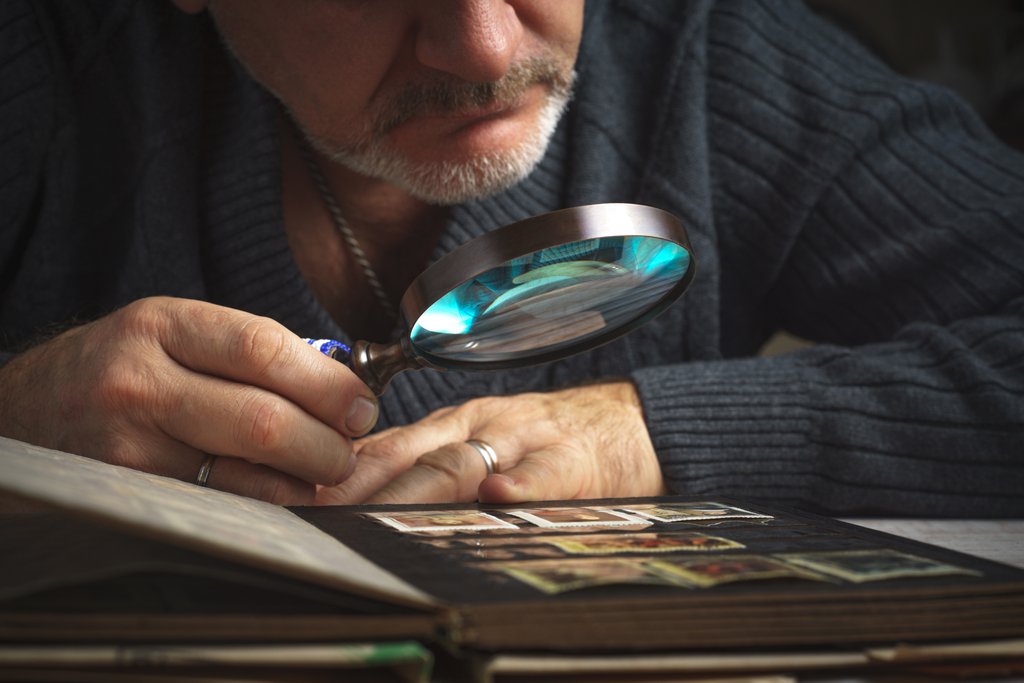This detailed color photograph features a late middle-aged or early elderly white man, characterized by his close-cropped white beard and dark mustache, closely examining a stamp album with a bronze-colored magnifying glass that has a blue lens. His deep cable-knit dark blue sweater and the wedding ring on his left hand are prominent. The magnifying glass is poised over a page within the album, suggesting his focused inspection of the large, white-framed, colorful stamps arranged in rows. The album, resting on a white table, reveals multiple scrapbooks underneath. The man's face, partially visible, shows his concentrated expression as he leans closely, with his chin, nose, and slightly reddened skin peeking into the frame. The surrounding scene provides an intimate view of a hobbyist deeply engaged in his stamp collection.